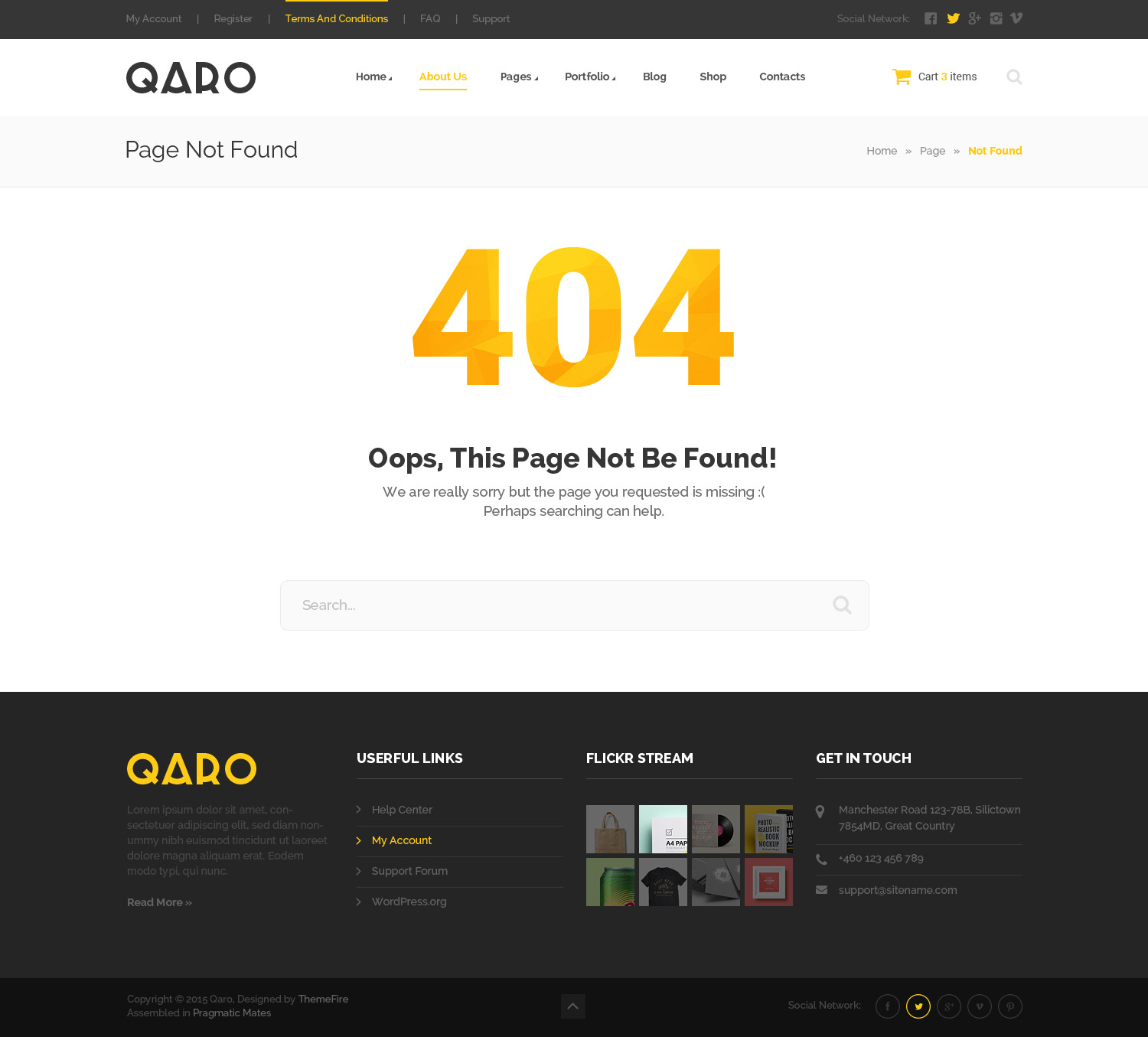In this image, we see a screenshot of a website spelled "Q-A-R-O," though the exact pronunciation is unclear. The page shown is a 404 error page, indicating that the requested page could not be found. Dominating the center of the page are large, yellowish-orange numbers "404." Below this, the text reads, "Oops, this page could not be found. We are really sorry, but the page you requested is missing. Perhaps searching can help." Beneath this message is a search box, inviting users to search for content on the site.

At the top of the page, several navigation links are visible: Home, About Us, Pages, Portfolio, Blog, Shop, and Contacts. Additionally, there is a shopping cart icon on the top right corner indicating that three items are in the cart, suggesting this site is an online shop. However, identifying specific products is difficult due to the presence of placeholder text ("lorem ipsum") and default template links, hinting that this might be a template or demo version of a shopping website.